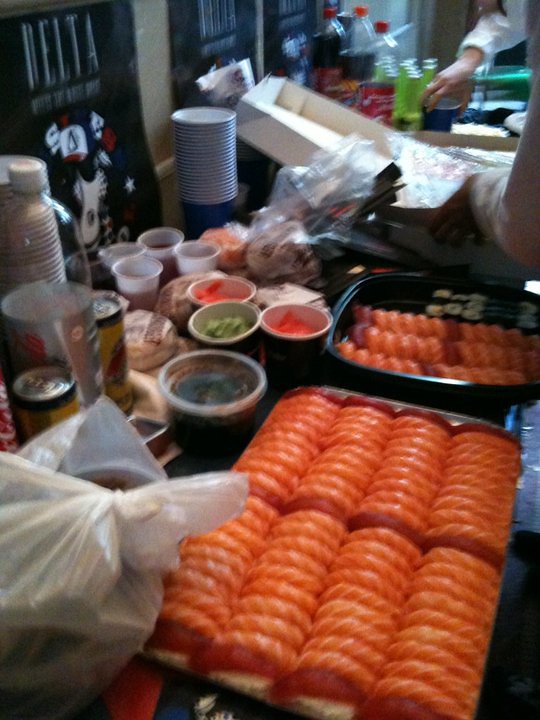This image captures a bustling scene that could be interpreted as an artist’s shelf or a setup for a casual buffet gathering. In the foreground, there is a box containing items that might be discs, coasters, or some fancy food items. Notably, there is an orange object that might be shrimp, segmented in square casings. Surrounding this are small white cups filled with muted shades of primary colored paints, which could also be interpreted as various foods—red, green, and dark sauces. Behind these, there is a plethora of food items including sushi platters prominently featuring tuna and darker red meat, and several yellow cans alongside a large Diet Coca-Cola bottle. In the background, a counter is cluttered with more food, soda bottles like Coca-Cola and Sprite or Mountain Dew, and an arm is visible holding a pizza box, while another hand clutching a blue cup is seen amidst tall containers of soda.